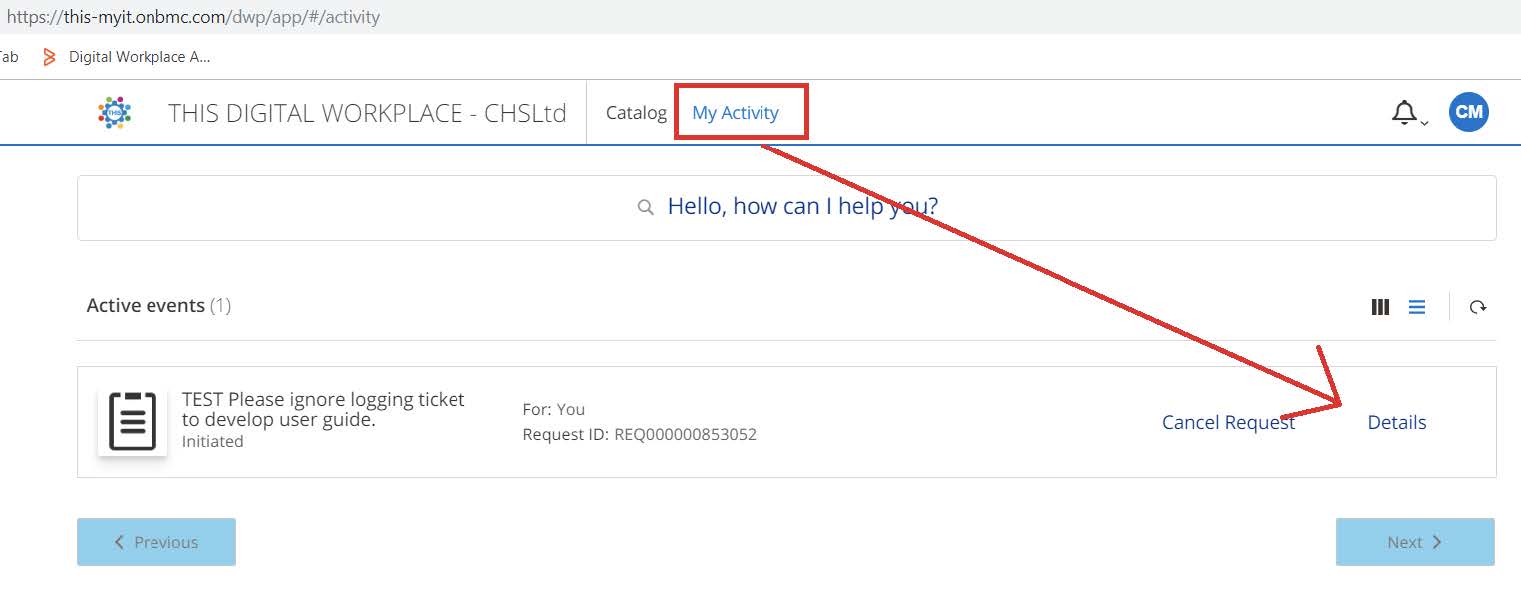A screenshot of a website displaying a specific section from the URL "https://this.myit.onbmc.com/DWP/APP/number/ACTIVITY". The page is part of the "AB Digital Workplace" under the "Digital Workplace / CHSLTD" catalog, and is specifically showcasing the "My Activity" screen. The "My Activity" section is highlighted with a red rectangle and an arrow pointing down to the "Details" of a specific activity.

In the main area of the screen, a prominent, circular "CM Hello, how can I help you?" search icon is visible. Below this, the section labeled "Active Events" is displayed with three menu bar options adjacent to it, as well as a refresh icon.

The highlighted activity within "My Activity" is marked by the label "Active Events." It includes a test event labeled "Please Ignore," indicating the initiation of a logging ticket to develop a user guide. The request ID for this activity is "REQ000000853052". There is an option to "Cancel Request" linked to this activity.

Towards the left side of the screen, a "Previous" bar is visible, while towards the right side, there is a "Next" bar, suggesting navigation options to browse through activities or events on this page.